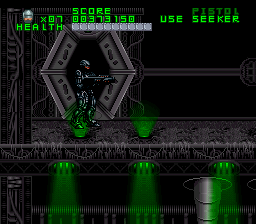In this small, square digital image from a computer game, the scene is predominantly black with vibrant neon green highlights. Central to the image, a character dressed in dark gray and black military gear, including a helmet, stands facing to the right, holding a rifle-like, semi-automatic firearm. The character's eyes are illuminated red, enhancing their stern appearance. 

They stand in front of an open hexagonal doorway, which features distinct green lights below, emanating rays upward and downward, illuminating the area. The floor beneath the character is marked with circular patterns, also radiating green light.

At the top of the image, green text displays various game stats and instructions. On the left, it reads "X 0 7" with "health" directly below it. In the center, it shows the score "00373150". On the right, it commands the player to "USE SEEKER".